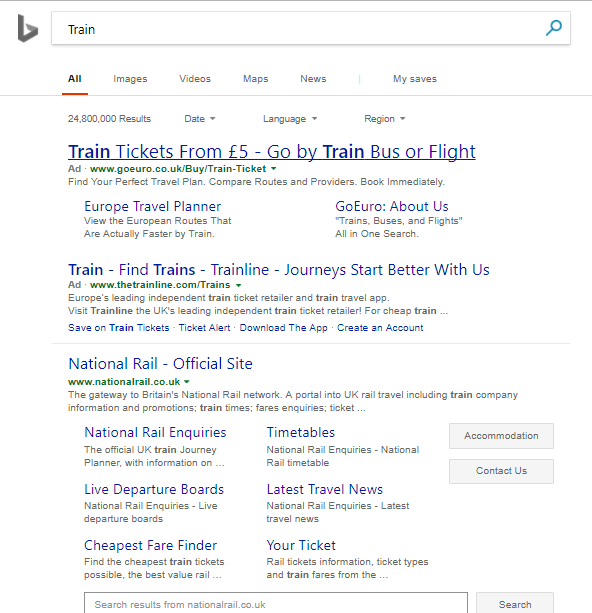The screenshot showcases search results from Bing, identified by the prominent 'B' logo in the upper left-hand corner, which appears in grayscale. Dominating the upper section is a large search field extended towards the right, accompanied by a blue magnifying glass icon on its right side. The search term entered is "train."

Directly beneath the search bar, a thin gray strip houses various categories—All, Images, Video, Maps, News, and My Saves. The 'All' category is highlighted in darker text with a red underline, indicating it is the selected option. 

The search results appear below the gray bar, starting with advertisements followed by organic links. The first ad, with prominent blue text, is for "Train tickets from five pounds," offered by goeuro.co.uk with the URL structure "/buy/train-ticket." The ad promotes finding perfect travel plans, comparing routes and providers, and booking immediately. The GoEuro planner option is mentioned on the left with an 'About Us' section on the right.

The subsequent ad is for "Train line," urging users to "find trains," with a tagline "Journey starts better with us." This advertisement is linked to thetrainline.com.

The first non-sponsored result is from the "National Rail - Official Site" at nationalrail.co.uk, shown in green text. This entry features multiple options: National Rail inquiries, live departure boards, cheapest fare finder, timetables, latest travel news, and ticketing information. Each option has a brief line or two of descriptive text underneath.

The layout is clean and structured, with various pertinent options for users seeking train-related information. Another search field is visible at the bottom of the page, encouraging further queries.